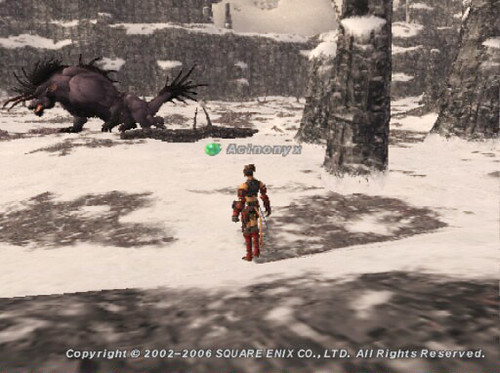The image is a sepia-toned screenshot from a video game set in a snowy, rocky landscape. The scene features small hills, rock formations, and a stone fence, all covered in a thin layer of snow. A gray dragon-like creature with spiky black hair on its head and tail is visible in the upper left corner. The focus is on a solitary figure in the center, dressed in a distinctive uniform with red boots and yellow accents, possibly wielding swords at their waist. There is some ambiguity in their appearance, suggesting they could be wearing body armor or even be a robot. Above the figure, the name "ACINONYX" is displayed. Along the bottom of the screenshot, it states, "Copyright 2002-2006, Square Enix Co., Ltd. All rights reserved."